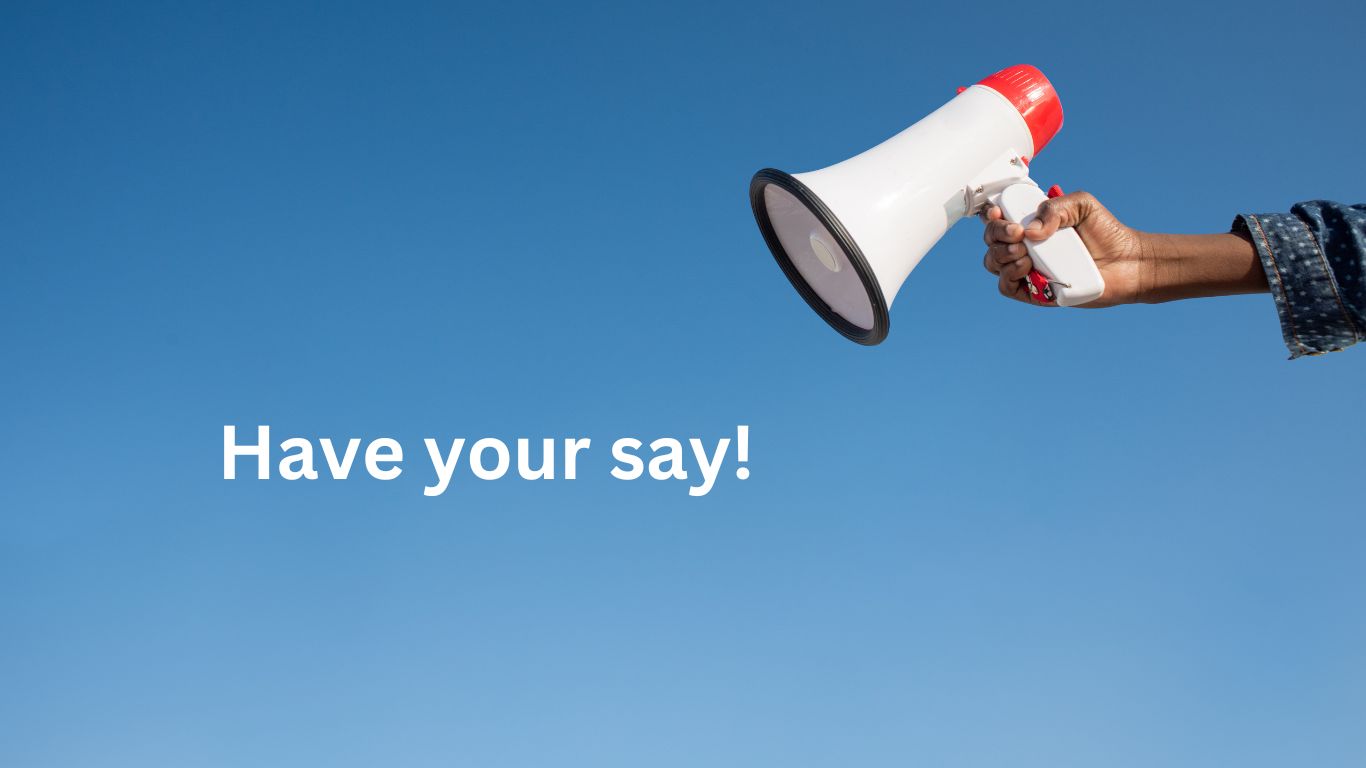In this image, an African-American woman holds a prominently featured white megaphone with red and black accents. The megaphone has red buttons and a red speaker section, while the rim of the broad end is black, likely made of rubber. She wears a blue, long-sleeved top, with the sleeves pushed back, and no nail polish on her fingers. Her right hand, visible only up to the wrist, clasps the megaphone, aiming it towards the center of the picture where the words "Have your say!" are boldly written in white Arial font. The background transitions from a darker blue at the top to a lighter blue at the bottom, creating an ombre effect that makes the white text stand out. Additionally, the megaphone extends towards the text, emphasizing a call to action.